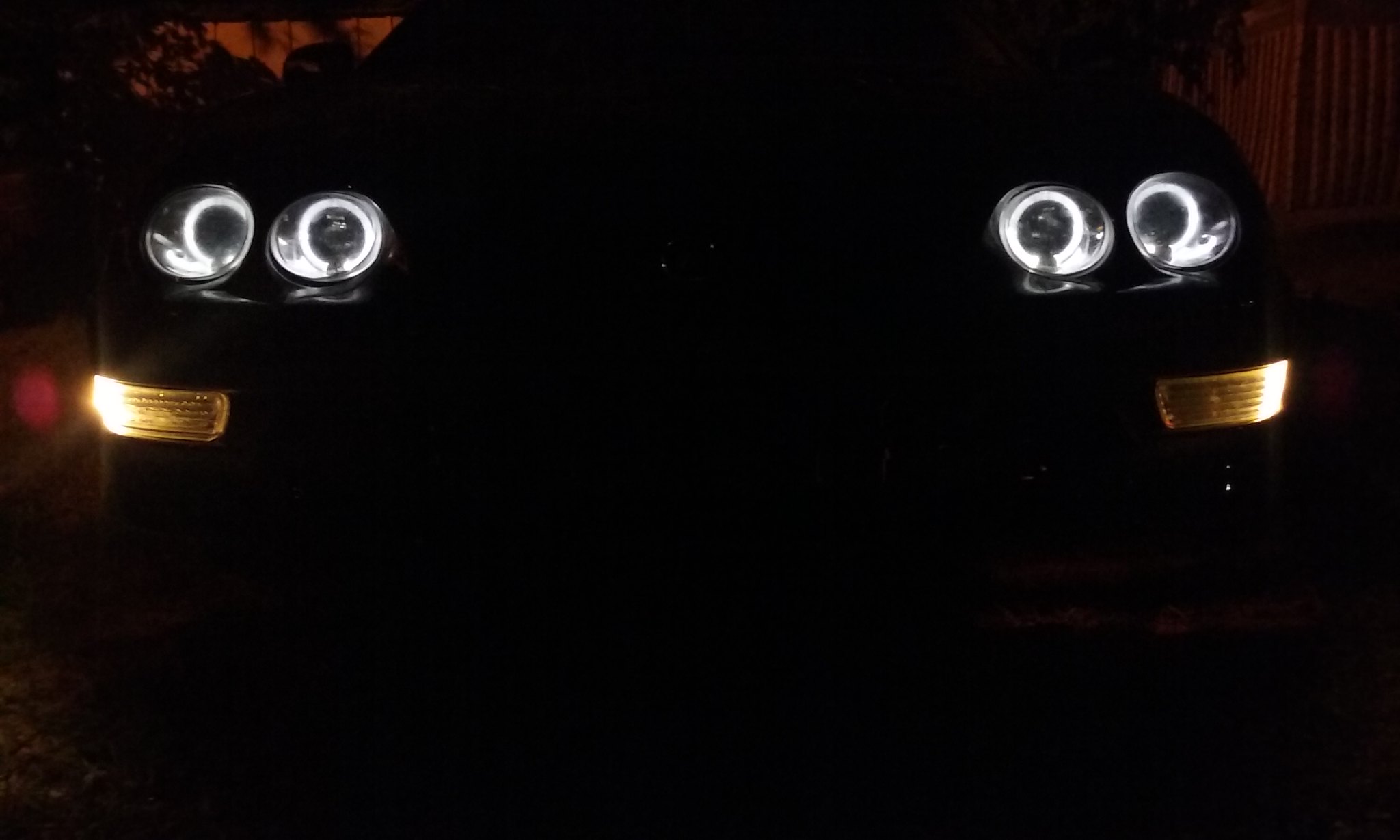In the photograph taken at night, a dark-colored car, possibly black, dominates the scene with its illuminated headlights and fog lights piercing through the darkness. The background is shrouded in the night, with vague outlines of trees and what seems to be a gate faintly visible. On both the left and the right front of the car, there are two large circular headlights emitting a bright white light, characteristic of halogen lamps, with a smaller black circle inside each light. Below these headlights on each side, two clear rectangular fog lights glow, further enhancing the car's outline. The headlights create an eerie effect, like two pairs of eyes staring out from the shadowy background. Although the car itself is silhouetted in black, its distinct, illuminated features provide stark details against the dark surroundings.